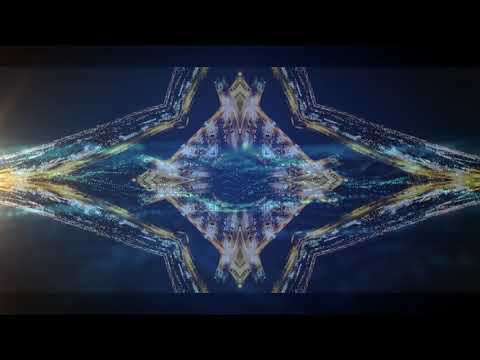The image features a dark blue fabric background with an abstract, geometric design at its center. The design prominently displays a vertical, white diamond shape. At the core of the diamond, there's a cobalt blue circle that somewhat resembles an eye. Surrounding this circle are intricate, smudged designs in various colors, including silver, gold, green, and black, creating an unfocused yet dynamic appearance.

Radiating from the diamond are four V-shaped points, effectively forming a cross or a four-pointed star. This star-like structure includes outlines in gray, blue, and yellow, which bleed into the surrounding dark blue background. The overall pattern carries a tie-dye aesthetic, with colors like yellow, white, and beige blending outwards in a messy yet intriguing fashion. The design is framed by white and cobalt blue trimming, which adds a sense of structure amidst the colorful smudges and blurred edges. On the left side of the image, light falls softly onto one of the star points, highlighting the textured fabric and adding depth to the complex, multi-layered pattern.